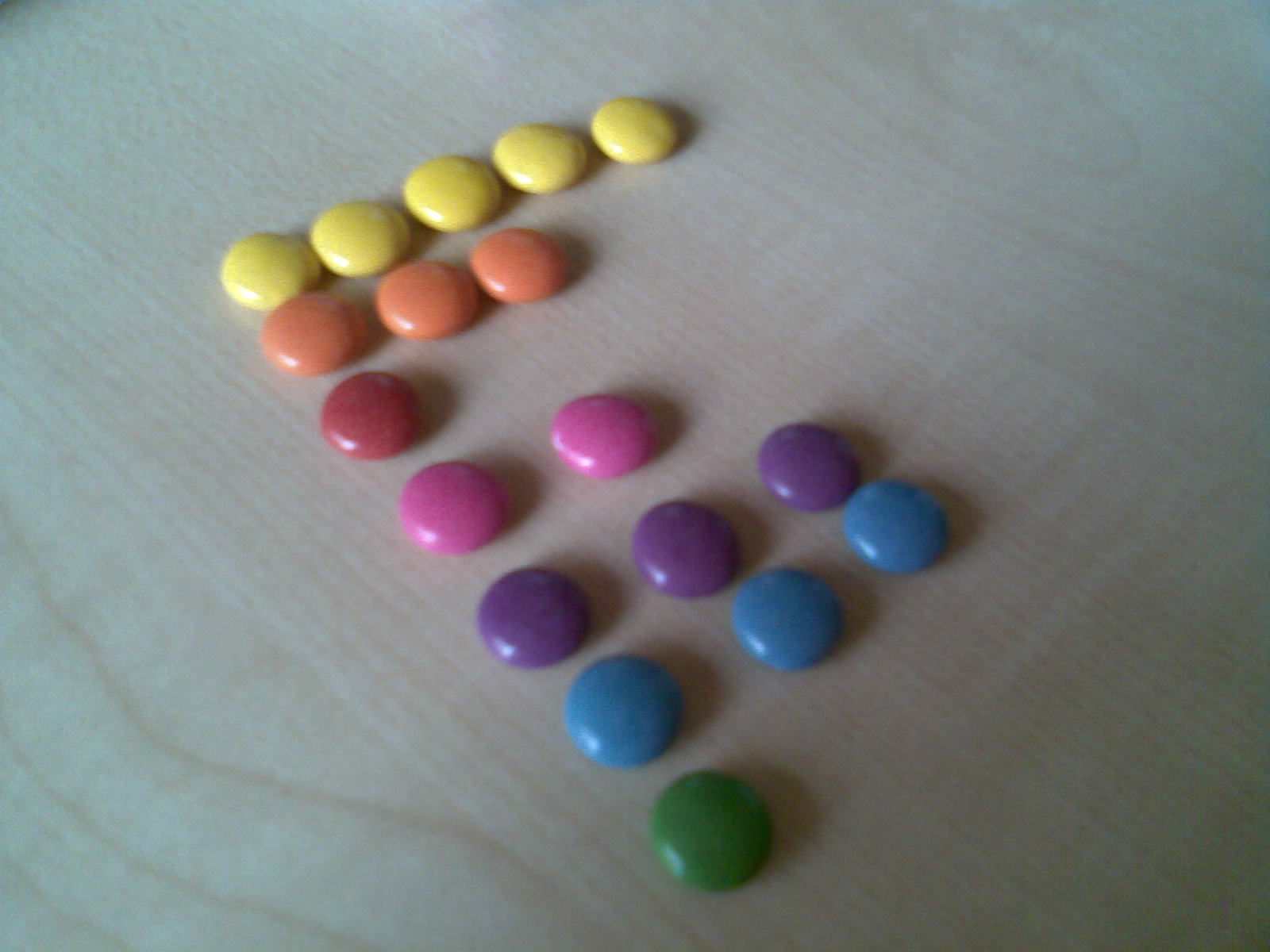This photograph showcases a neatly arranged formation of multi-colored, candy-coated chocolates resembling Skittles, placed on a slightly out-of-focus wood grain surface. At the top of the arrangement, there is a row of five yellow candies. Below this, a sequence of three orange or salmon-colored candies is aligned. Further down, a single red candy is positioned, followed by two light pink ones beneath it. The next row features three purple candies, succeeded by a line of three medium blue candies. At the bottom of the formation, a solitary green candy appears. Collectively, the candies are set in straight rows and columns, creating an organized yet abstract design that could suggest the shape of a letter or simply a deliberate pattern.